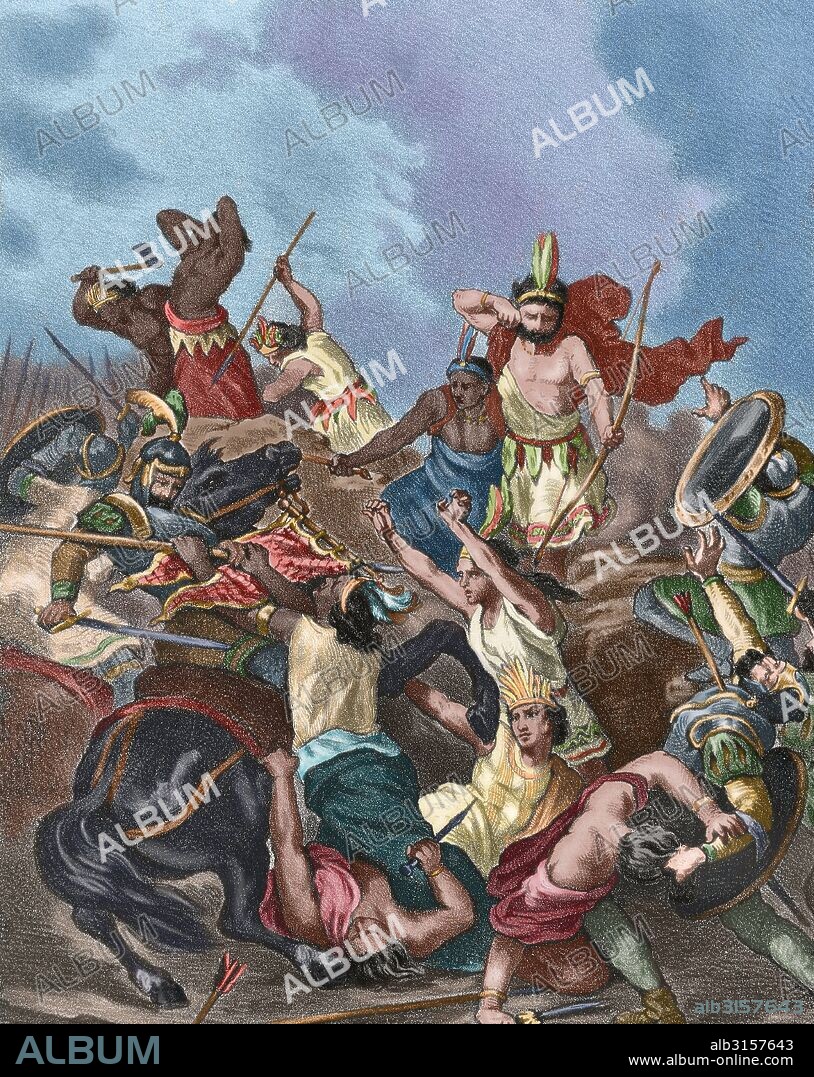This vertically aligned rectangular image appears to be an album cover. The word "album" is diagonally printed throughout the image in a mix of gray and white text. At the bottom, there is a black border; on the lower left, the word "album" is printed in green, and on the lower right, there are numbers ("ALB 3157643"), along with the web address "www.album-online.com" in white text.

The main scene is a chaotic and detailed depiction of an ancient battle. Numerous warriors, dressed in robes of varying colors—white, blue, and red—engage in intense combat with spears, swords, and bows and arrows. One man, in particular, stands with his hands up as if surrendering, while another points a spear at a helmeted individual. A warrior on the right stretches back a bow, ready to shoot. An imposing figure rides a black horse, brandishing a sword and pointing towards another combatant. Amidst the fray, a man in a red robe lies on the ground, aiming a large knife at an opponent dressed in yellow. The background of the scene blends dark and light blue hues with patches of gray, resembling a sky transitioning from day to night.